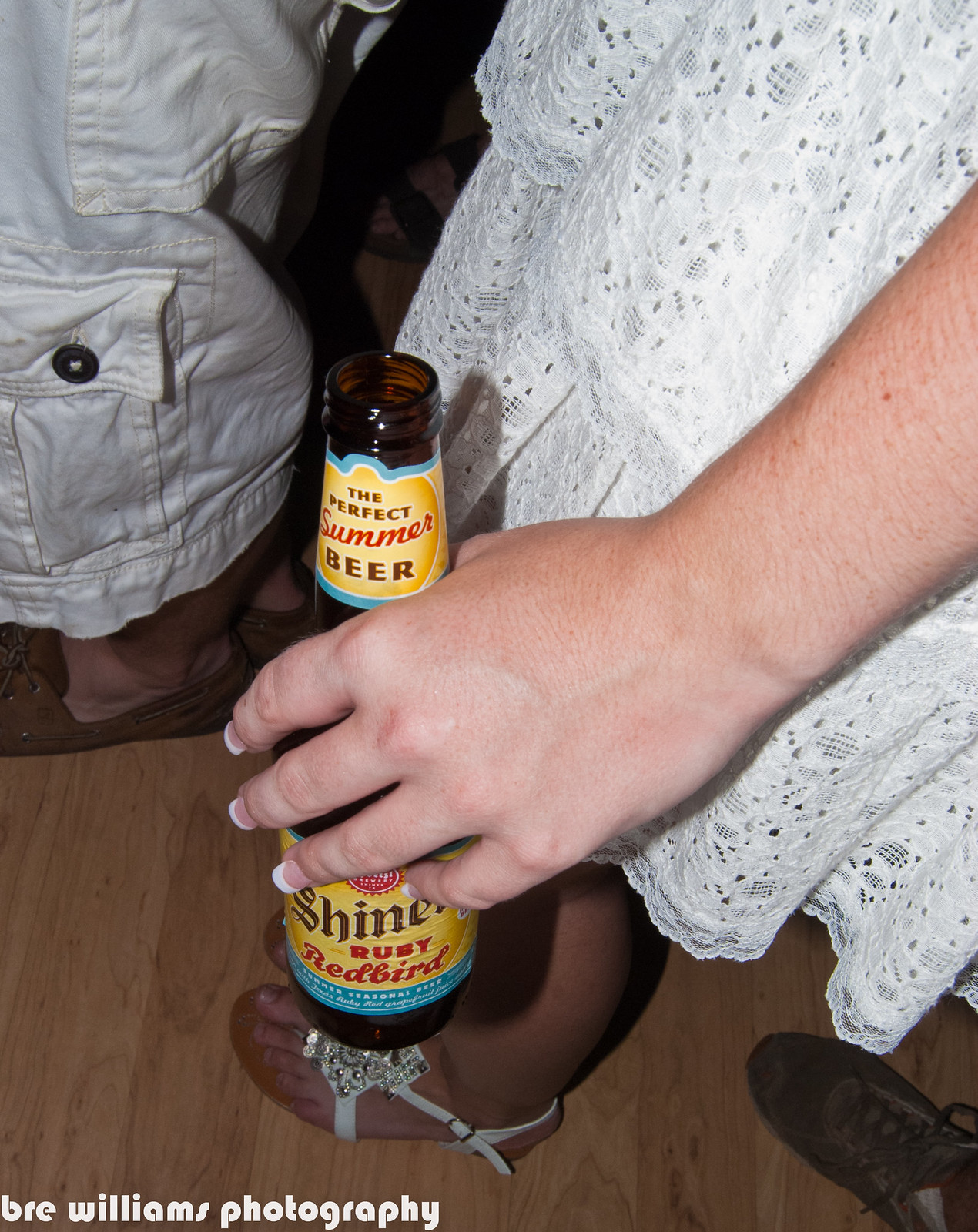In the photograph taken by Bree Williams Photography, two individuals stand closely together, captured from the torso down. The scene highlights the intricate details of their attire and accessories. One person is dressed in beige cargo shorts paired with loafers, providing a casual contrast. The other individual dons a delicate white lace dress and eye-catching white jeweled sandals, perfectly complemented by a chic French manicure. In her hand, she holds a brown bottle of Shiner's Perfect Summer Beer, specifically the Ruby Redbird flavor, distinguished by its yellow label with red lettering. The professional touch of the photography is signified by the discreet white font in the bottom left-hand corner of the image, marking the creator's name: Bree Williams Photography.